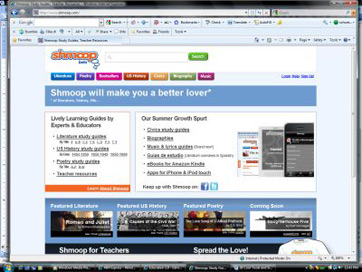This image is a blurry screenshot of a computer’s browser window capturing a website. The browser interface shows multiple open tabs at the top, with a gray strip, a white address bar, and various toolbars below it. The website itself features an old Google search bar at the top, various icons, and a predominantly white content area set against an orange background.

Near the top, there’s a white search bar followed by a green and white search bar. Below that, a series of vibrant submenus are visible in colors such as blue, purple, pink, rusty orange, gold, and green, each with white text that is difficult to decipher.

Further down, a blue box displays the white text "SHMOOP will make you a better lover," with smaller white text below it. Adjacent to this, there is another white box with black text that appears to contain guides, although the exact content is hard to read.

On the right-hand side, the text "Our summer growth spurt" is visible along with several clickable black links. There are also various thumbnails and icons, including those for Facebook and another unnamed blue social media platform, alongside visuals of smartphones and tablets.

The lower part of the screenshot includes additional images with white text indicating topics like U.S. history and literature. A black bar reads "Sham Pop for teachers and spread the love," and more tabs can be seen at the bottom of the window.